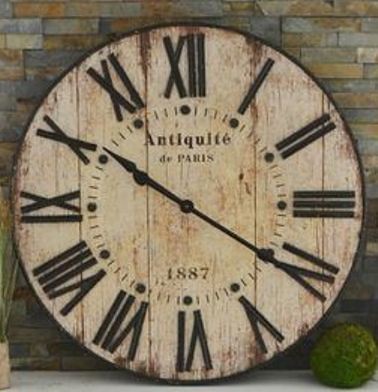A large, intricately designed wooden clock is the focal point of this image, set against a backdrop of gray brick. The clock, which seems to be either propped up against a surface or featured in a close-up shot, boasts a rich wood grain texture. Its face is adorned with black Roman numerals, and pairs elegant black hands indicating the time to be approximately 10:20. At the top of the clock face, the inscription "Antiquite de Paris" stands out, adding a touch of old-world charm. Towards the bottom, the year "1887" is prominently displayed. A small bush peeks into the frame from the lower right corner, providing a hint of natural greenery in the scene.